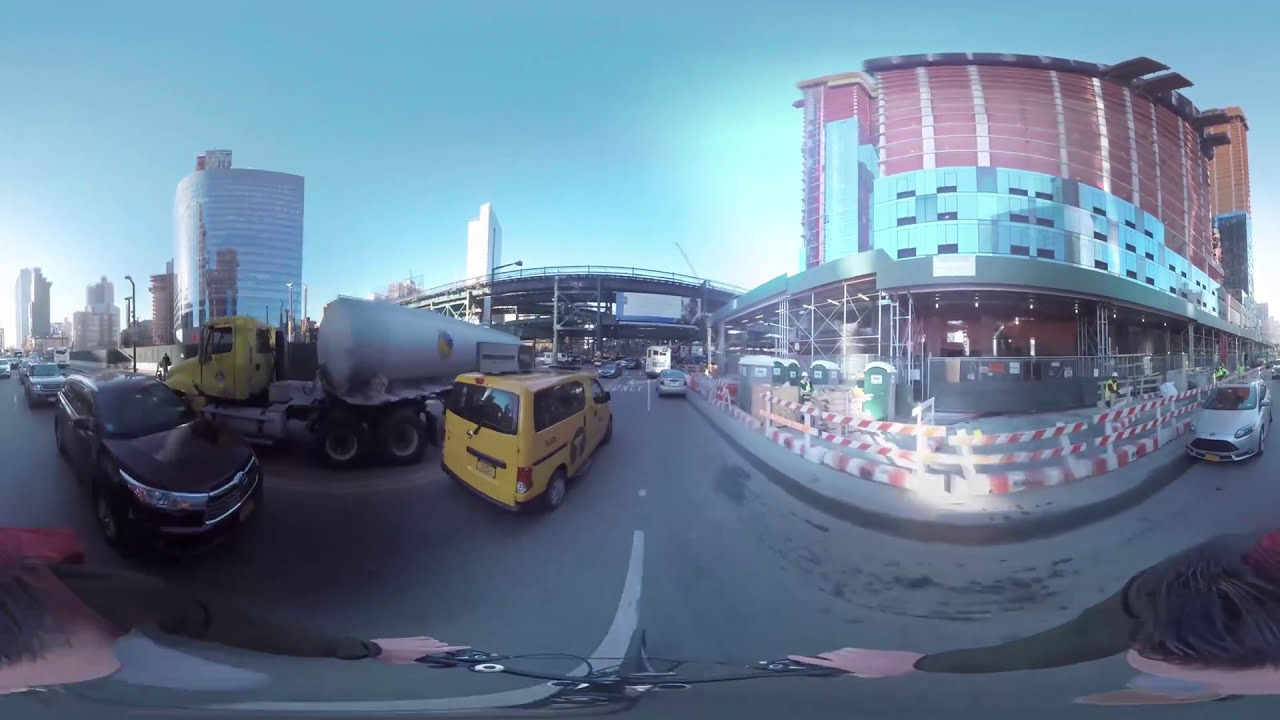The image, captured from a bicyclist's perspective, likely using a helmet-mounted or handlebar camera, showcases a bustling city street through a fisheye lens. The bicyclist, wearing a dark long-sleeved shirt, grips the bike handlebars with both hands, visible at the bottom of the image. Heavy traffic surrounds him, including a yellow minivan (possibly a taxi) and a black sedan or crossover vehicle. A large tanker truck with a yellow front is making a right turn at an intersection ahead. On the right side of the street, a red and glass rounded building under construction is visible, surrounded by scaffolding, barricades, and several porta potties. The surrounding environment includes multiple 10 to 15 story glass buildings and a tall skyscraper in the distance. The fisheye effect distorts the scene slightly but captures the clear daytime sky and the dense urban setting.